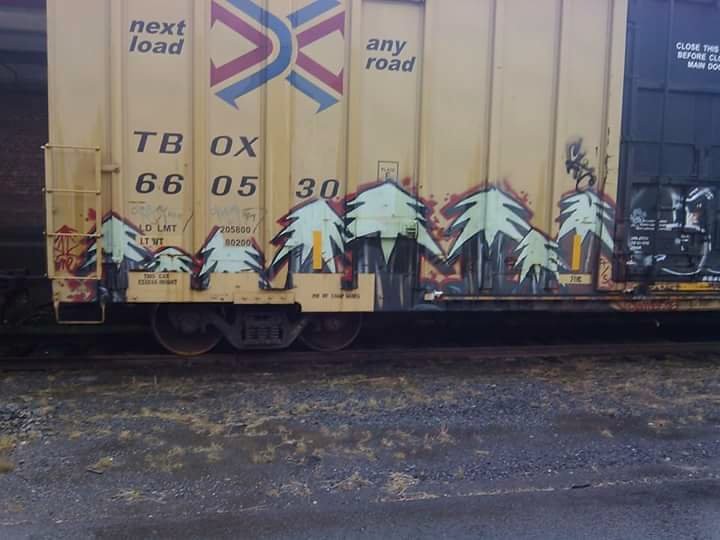In this photograph, a detailed side profile of a cargo train car is captured. The central focus is a yellow boxcar featuring vivid blue and red criss-crossing arrows. Prominently displayed on the car are the bold black letters “Next Load, Any Road” along with the identifier “TBOX 6605 30”. The left side of this boxcar showcases a short four-rung metal ladder leading to the platform, with the wheel carriage and track visible beneath it. The ground beneath the train is scattered with rock and brown grass, interspersed with standing water.

The side of the car is adorned with graffiti depicting black-outlined fir trees filled in with blue, varying in height from six inches to a couple of feet, totaling eight distinct trees. Adjacent to this boxcar, a portion of a second dark-colored car is visible, marked with regulatory instructions but mostly covered in indecipherable white graffiti. The entire scene is set against a backdrop of black cement, highlighting the industrial atmosphere of the train yard.